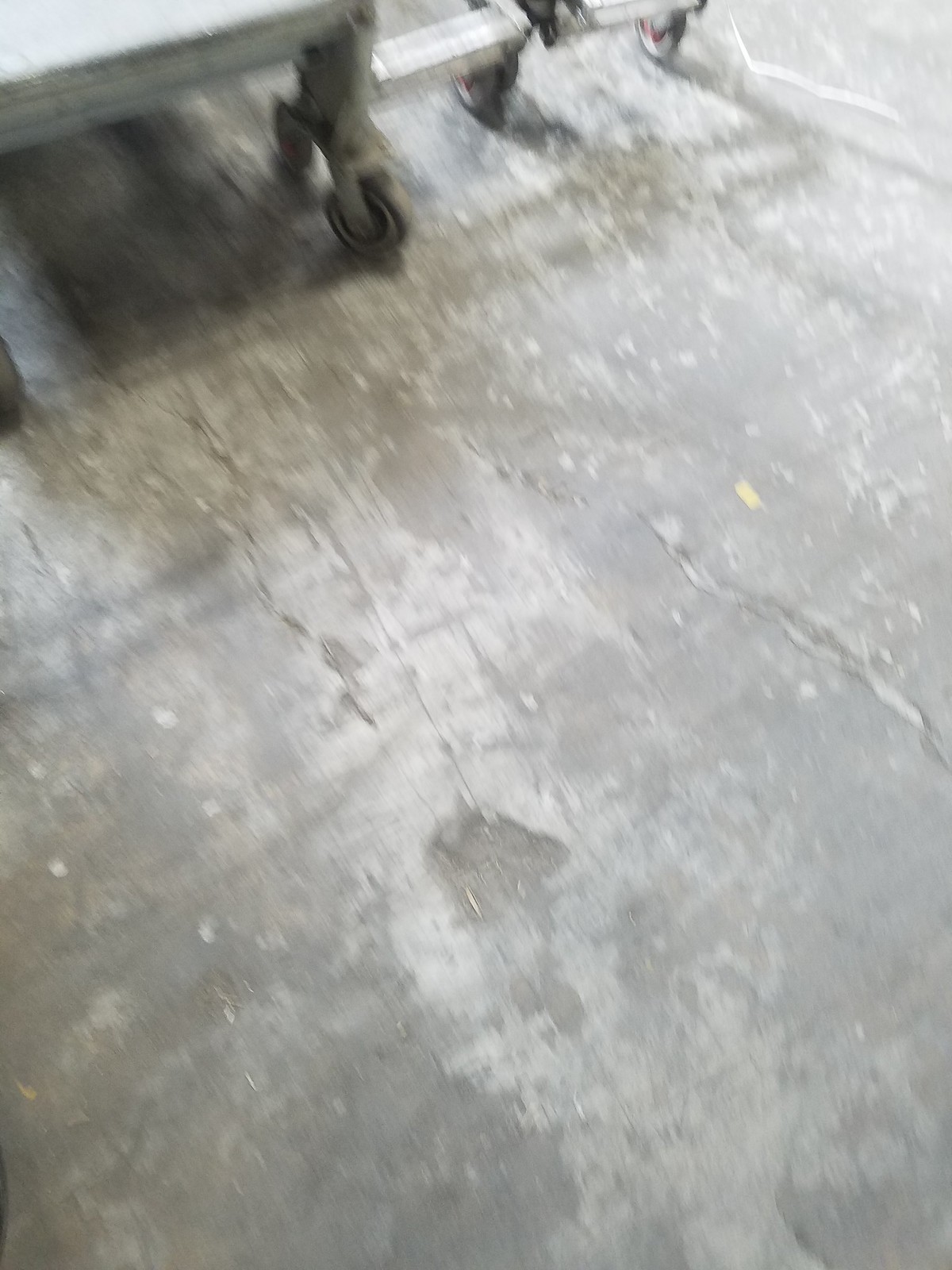This image captures an aged, heavily worn concrete floor, probably within an industrial workspace such as a garage or warehouse. The gray cement surface is marred by numerous cracks, chips, dings, and a visible hole in the center, suggesting extensive use and wear over time. The floor surface appears discolored and could benefit from cleaning. Along the top edge of the photo, slightly cut off, are several heavy-duty metal trolleys or push carts with thick metal legs and black wheels. The shadow beneath these carts hints at the depth of their structure. The good lighting in the image indicates it might have been taken on a well-lit day, potentially outside or in a space with ample natural light.